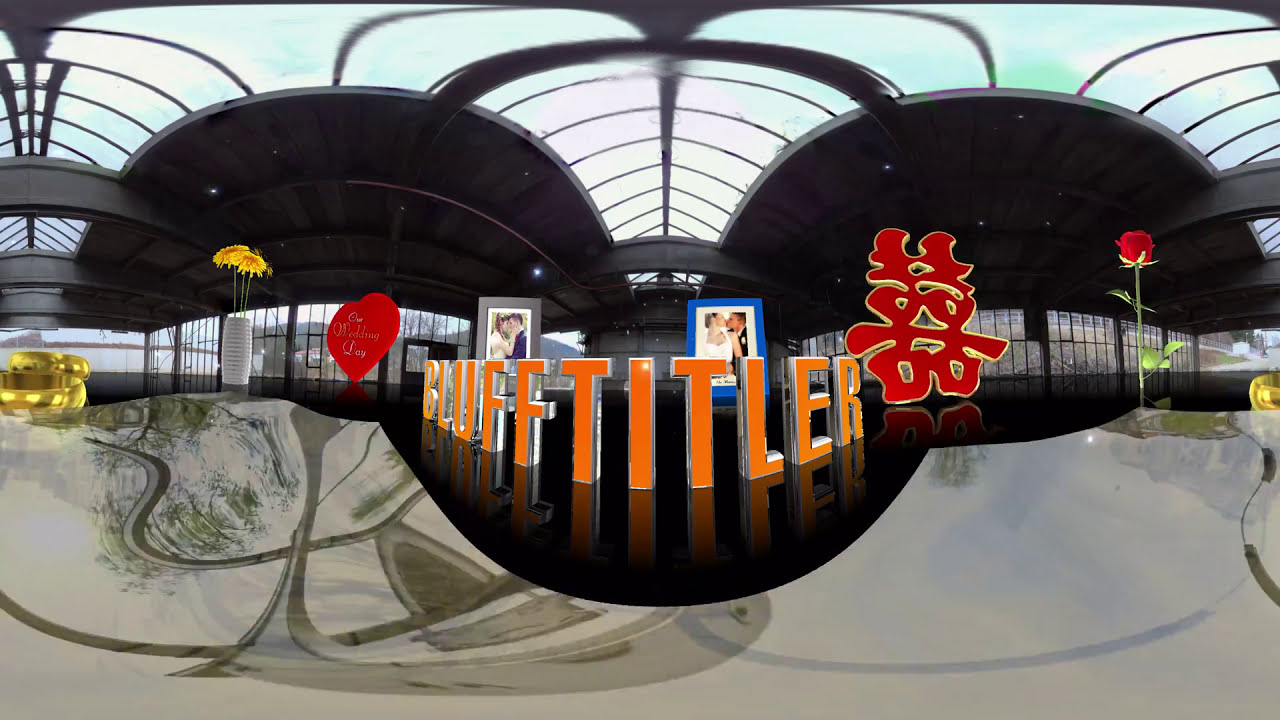In this vibrant and detailed photograph, a captivating and artfully arranged scene grabs the viewer's attention. Dominating the center are large, three-dimensional orange letters that spell "Bluff Titler" in a semi-circle. Just behind these letters, two framed photographs are prominently displayed, portraying a wedding couple—in one image, they are dancing, while in the other, they share a kiss. 

To the left of this central focal point, a red heart with the text “Our Wedding Day” adds to the romantic ambiance, accompanied by a white flower vase filled with bright yellow flowers. Further to the left, gold ornamental details catch the light, possibly a chair or a decorative object. On the far right, Asian characters in red add an exotic touch next to a vertical red rose with green leaves. 

The backdrop of this setup features blackish-gray, curved metal structures that resemble the interior ceiling of a modern building, punctuated by open windows that allow natural light to pour in. Below, a sophisticated gray stone or glass surface with artistic wavy patterns adds a final touch of elegance to this meticulously crafted scene, which collectively evokes the joyous celebration of a wedding day.